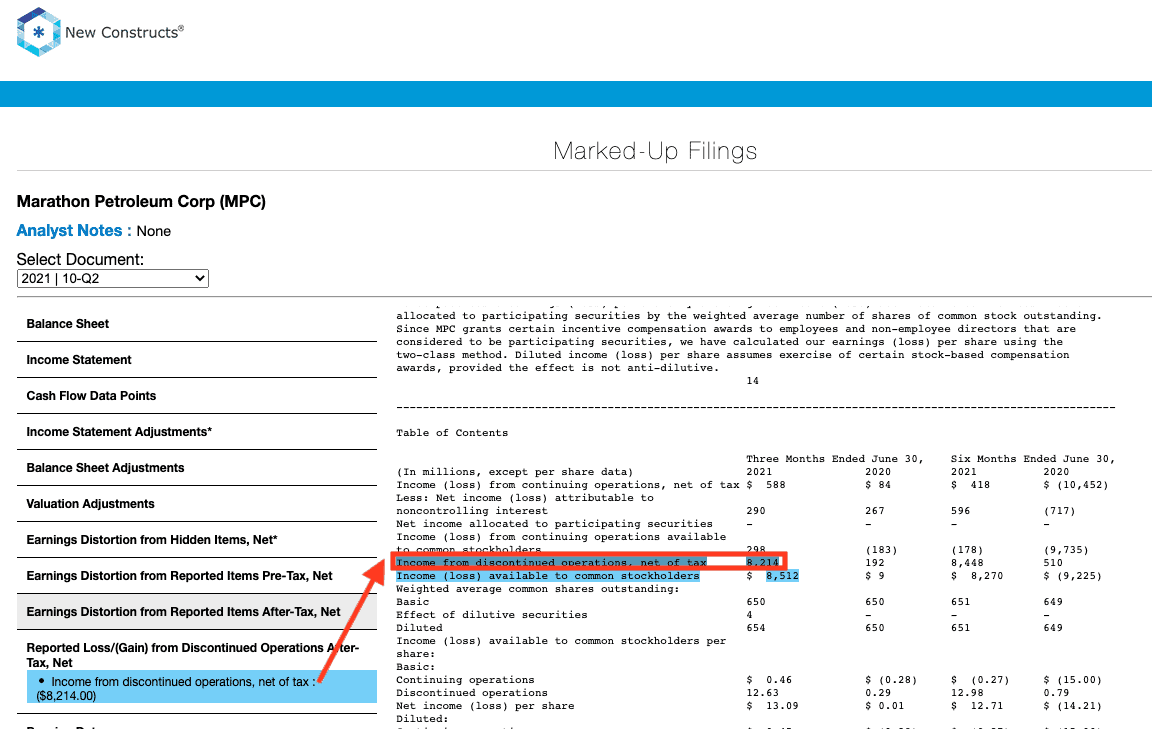The image showcases a webpage titled "New Constructs," featuring a registered trademark symbol next to the "Constructs" label. Central to the branding is a geometric logo, blending hexagonal and diamond shapes with multicolored line segments varying in shades and intensities of blue, with a snowflake design at its core. Below the logo, a broad, horizontal blue bar stretches across the image, separating the "New Constructs" title from the phrase "Marked Up Filings," which is center-aligned beneath the bar.

On the left margin of the page, the text "Marathon Petroleum Corp (MPC)" stands out in bold, black font. Just below, in blue text, it states "Analyst Notes: none." Following this, the line "Select a Document" is accompanied by a drop-down box currently set to the year 2021 and "Q2" (Quarter 2), suggesting the option to choose different years or quarters.

Further down, the page lists a series of financial document labels in a structured format, including "Balance Sheet," "Income Statement," "Cash Flow Data Points," "Income Statement Adjustments," "Sheet Adjustments," "Evaluation Adjustments," "Earning Distortion from Hidden Items, net," "Earnings Distortion from Reported Items," "Pretax Distortion," "Post-Tax," "Reported Loss and Gain from Discontinued Operations." Additionally, a highlighted blue section notes "Income from Discontinued Operations, Net of Tax: $8,214," with a corresponding arrow pointing towards relevant details.

To the right, the detailed table includes various financial metrics and statements, mentioning figures like losses and millions. The specific entry "Income from Discontinued Operations: $8,214," and "Available to Accountable Stockholders: $8,412" are highlighted. The table further breaks down financial data across different time periods, including a three-month ending on June 30th and a six-month ending on June 30th, with information spanning from 2021 to 2022.